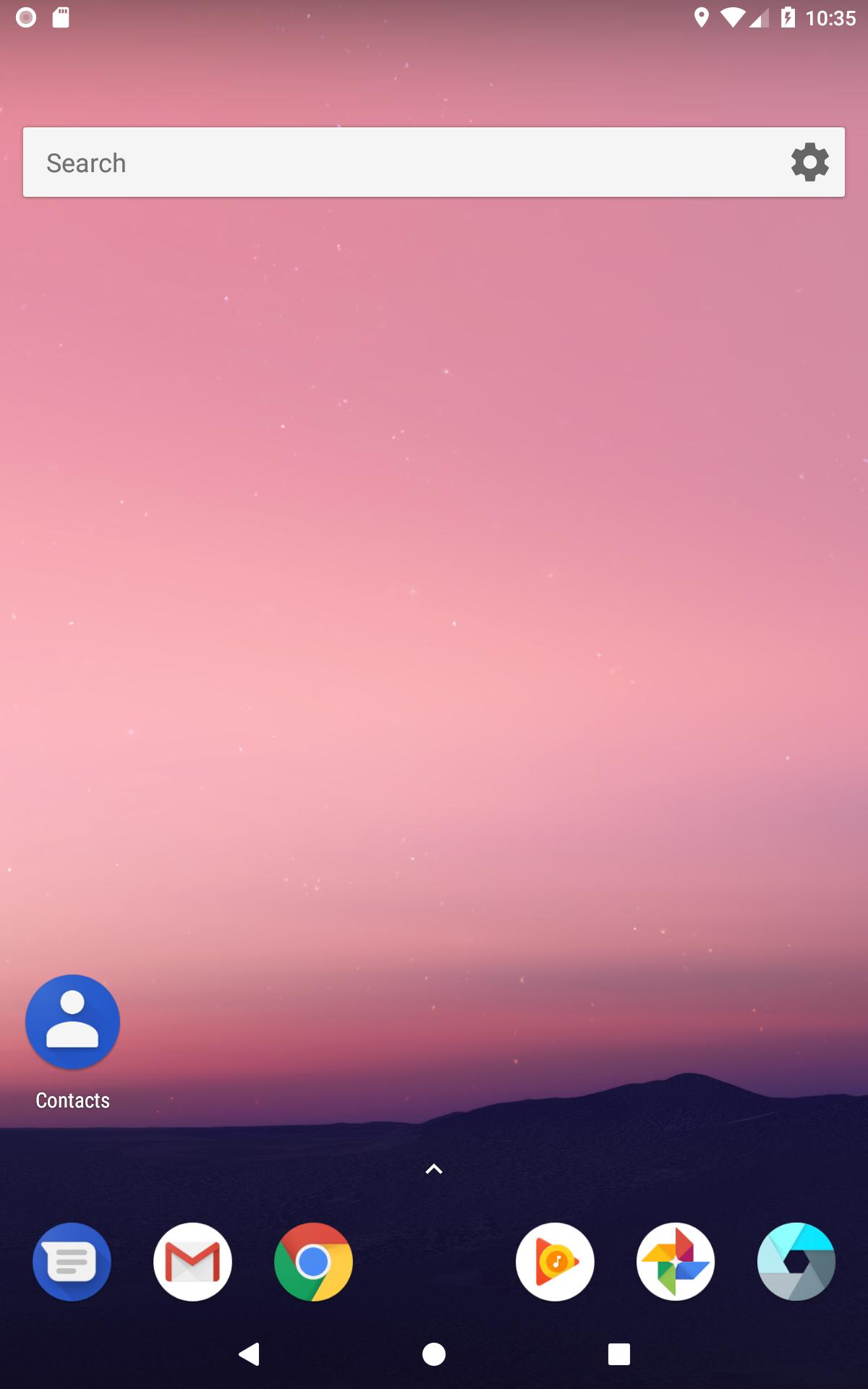The image captures the screen of a smartphone, beautifully illustrating various elements in crisp detail. At the top of the screen, multiple status indicators are visible, including Wi-Fi signal strength, battery level, and the current time. Just below these indicators lies a search box labeled "search," accompanied by a settings gear icon in gray.

The main portion of the screen showcases a visually striking background, featuring a warm, reddish hue reminiscent of a sunset, scattered with a myriad of stars. This background sets the stage for a variety of functional buttons and icons.

Prominently displayed is a “Contacts” button, symbolized by a blue icon with a white outline of a person. Lower on the screen, several other app icons are laid out, each distinct in color and design. There is a messaging icon with a blue background and white text, a Gmail icon characterized by a red and white envelope, and the Chrome browser icon in its iconic green, red, yellow, and blue palette.

Additional app icons add to the diversity of the display. One icon sports a white background with a red and yellow center, while another features a combination of yellow, red, blue, and green elements within a white circular background. A different circular icon is noticeable with its light blue and gray shades.

At the bottom of the page, essential navigation buttons are neatly aligned - a white back arrow, a circle symbol which typically represents the home button, and a square, all also in white. This well-organized array of icons and buttons creates a comprehensive and highly functional smartphone interface.